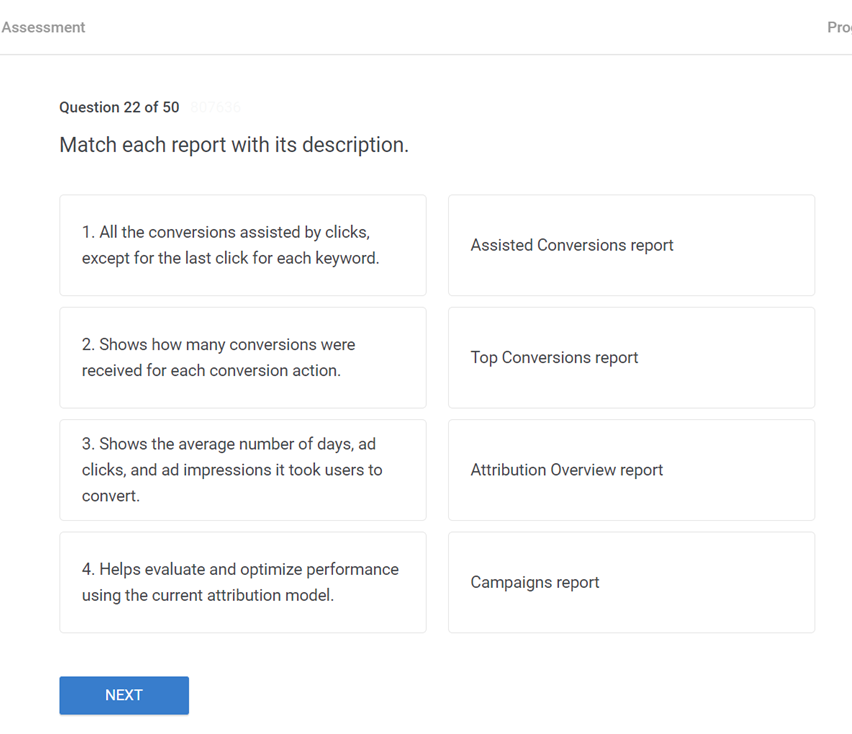The image depicts a section of an online assessment interface. The interface is divided into two sections with the word "Assessment" on the left and "Pro" on the right. The current question, number 22 out of 50, indicates the assessment is well underway. The question prompts users to "Match each report with its description," suggesting a multiple-choice format.

The question and corresponding answers are displayed within a white box outlined in light gray. The descriptions to be matched with their respective reports are as follows:

1. "All the conversions assisted by clicks except for the last click for each keyword."
2. "Shows how many conversions were received for each conversion action."
3. "Shows the average number of days, ad clicks, and ad impressions it took users to convert."
4. "Help evaluate and optimize performance using the current attribution model."

The options to match these descriptions with are:
- Assisted Conversions Report
- Top Conversions Report
- Attribution Overview
- Campaigns Report

At the bottom left of the interface, there is a "Next" button, a solid blue box with the word "Next" in white, indicating progression to the next page of the assessment. The overall design of the website appears minimalist, with a primarily black and white color scheme.